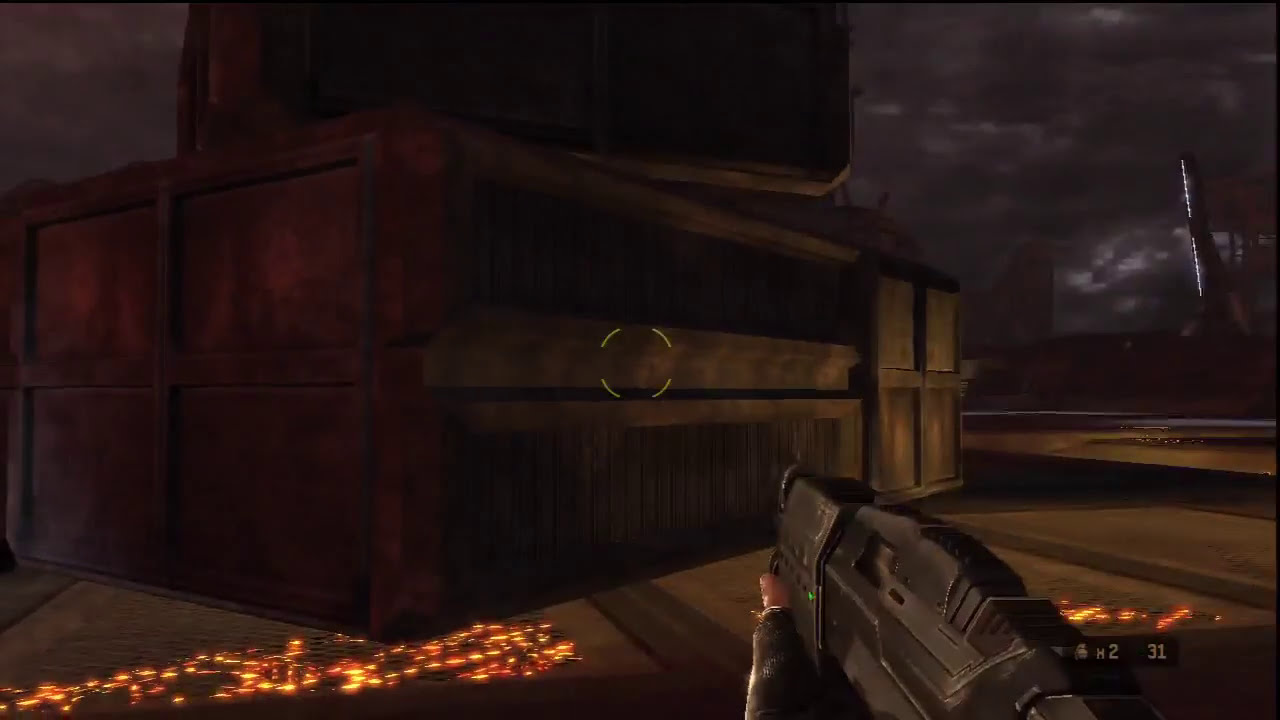The screenshot captures a first-person shooter video game interface. The player is wielding a futuristic, metallic-looking gun, pointed slightly to the left, with a fingerless-gloved thumb visible gripping the front barrel. The game's minimalist UI features a central reticle formed by four curved lines creating a square shape and a semi-translucent rectangle in the bottom right displaying an icon of a grenade with the indicator "x2" and the ammunition count "31". The scene showcases a large, tan-colored, metallic box that spans nearly the entire width of the image, rotated about 45 degrees counterclockwise. The environment suggests a dark, stormy atmosphere with a cloudy sky overhead. The foreground glows with a golden, firelike patch, particularly noticeable in the bottom left corner, hinting at a sparkly effect resembling fire on the grated floor beneath and to the right of the box. The player appears to be aiming at the box, possibly indicating a target symbol centered on it.